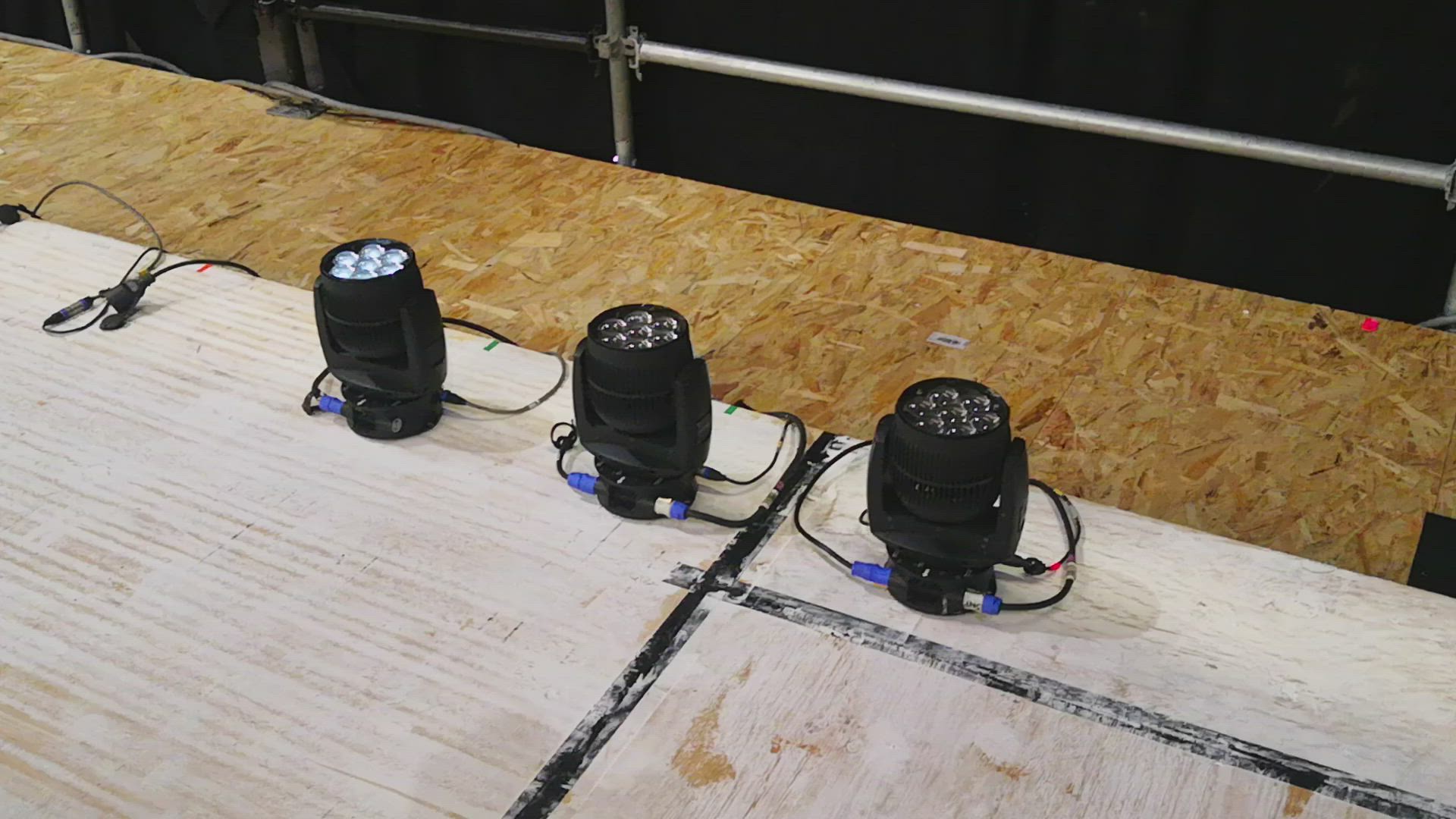This close-up photograph, taken in an interior setting possibly resembling a stage or workshop, features a detailed view of three round lamp lights. The image is in landscape mode, with a black backdrop held up by silver metal railings cutting off at the top of the frame. Below the railings, there is a natural wooden board, and atop that is a roughly painted white wooden board. Along the edge of this white board, connecting to the natural wood, sit three distinct lamp lights. Each lamp has a black base and a bubble-like clear lens at the top, likely containing powerful bulbs. Visible are multiple wires, some of which loop around and might connect underneath the plywood, implying these lamps are adjustable and can be tilted. The lamps appear identical in size and configuration, with one on the left already lit up. Descriptive details also include mentions of a cork-like table surface with light brown and cream colors, adding to the complex and intriguing composition of the image.